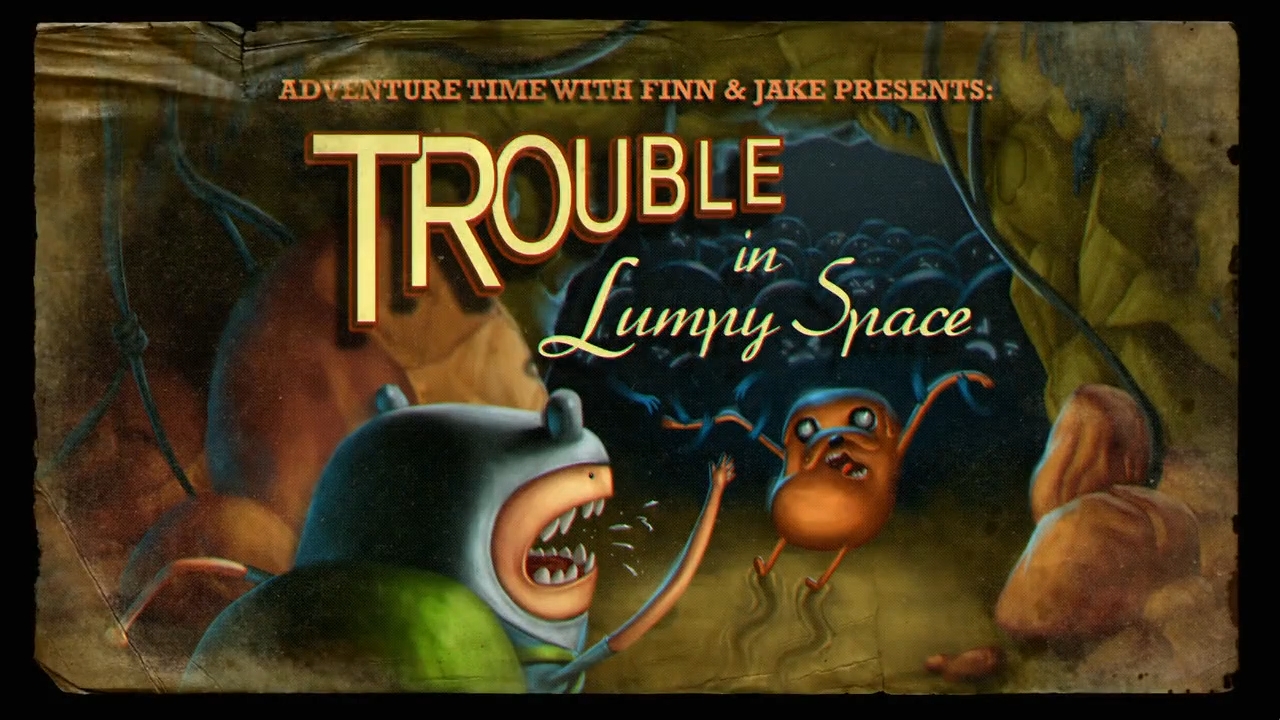In this detailed illustration, we see an eerie scene set in front of a spooky cave surrounded by brown boulders with green vines growing above the arched opening. At the forefront of the image, there's a gray-headed, green-bodied insect-like monster with gray beady eyes on its head, a mouth outlined in light tan with sharp white teeth, wide open and spewing something. Facing this creature, there is a brown peanut-shaped character with a dog-like nose, dark eyes, and an open mouth displaying sharp teeth and a tongue, extending long, skinny arms and legs. In the background, the dark entrance of the cave is ominously lit with beady eyes peering out toward the viewer. The sky above them features bold, colorful text that reads "Adventure Time with Finn and Jake presents Trouble in Lumpy Space," with "Trouble" prominently highlighted in yellow and red underline. The scene captures a moment of heated confrontation between the two main characters, adding an intense and adventure-filled vibe to the poster.